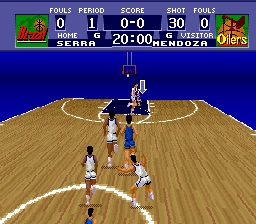The image is a pixelated, 8-bit style screenshot of a basketball video game, resembling an old television or PlayStation game. The court has a brownish wood grain texture with white outlines, including a visible white circle in the bottom left corner. The background is a deep blue with lighter blue shading.

At the top of the screen, a scoreboard indicates it’s the first period, with the score at 0-0, 30 shots taken, 0 fouls for both teams, and a timer set to 20 minutes. The left side is labeled "Home" for Brazil, and the right side is "Visitor" for the Oilers, although there is some ambiguity in the names mentioned ("Sara Mendoza" and another, less clear name).

The game features players in white and blue jerseys. In the foreground, there's a mix of figures: one with dark skin in a white uniform and white socks running, another in a white uniform pushing to the left, and other figures in white and blue uniforms. Further down, a basketball hoop hangs from the ceiling in front of a blue-painted area marking the paint zone and the three-point line.